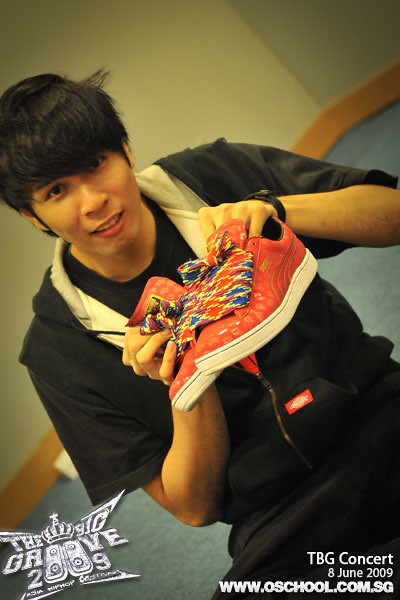In this photograph, a young Asian man, possibly a teenager or in his early twenties, is holding up a pair of distinctive red Puma sneakers for the camera, displaying them proudly. He wears a black Dickies hoodie with white lining over a black t-shirt and matching black pants. The young man, with shaggy black hair and bangs that cover his forehead, has a slight smile on his face. The sneakers he's holding feature thick shoelaces with a striking, multicolored diamond pattern in blue, red, and yellow, resembling almost a Native American design. The photo is taken with the camera tilted, so the blue floor and white walls with a light brown baseboard appear askew. There are two watermarks on the image: "The Groove 2009" at the lower left-hand side and "TBG Concert 8 June 2009 www.oschool.com.sg" at the bottom right.